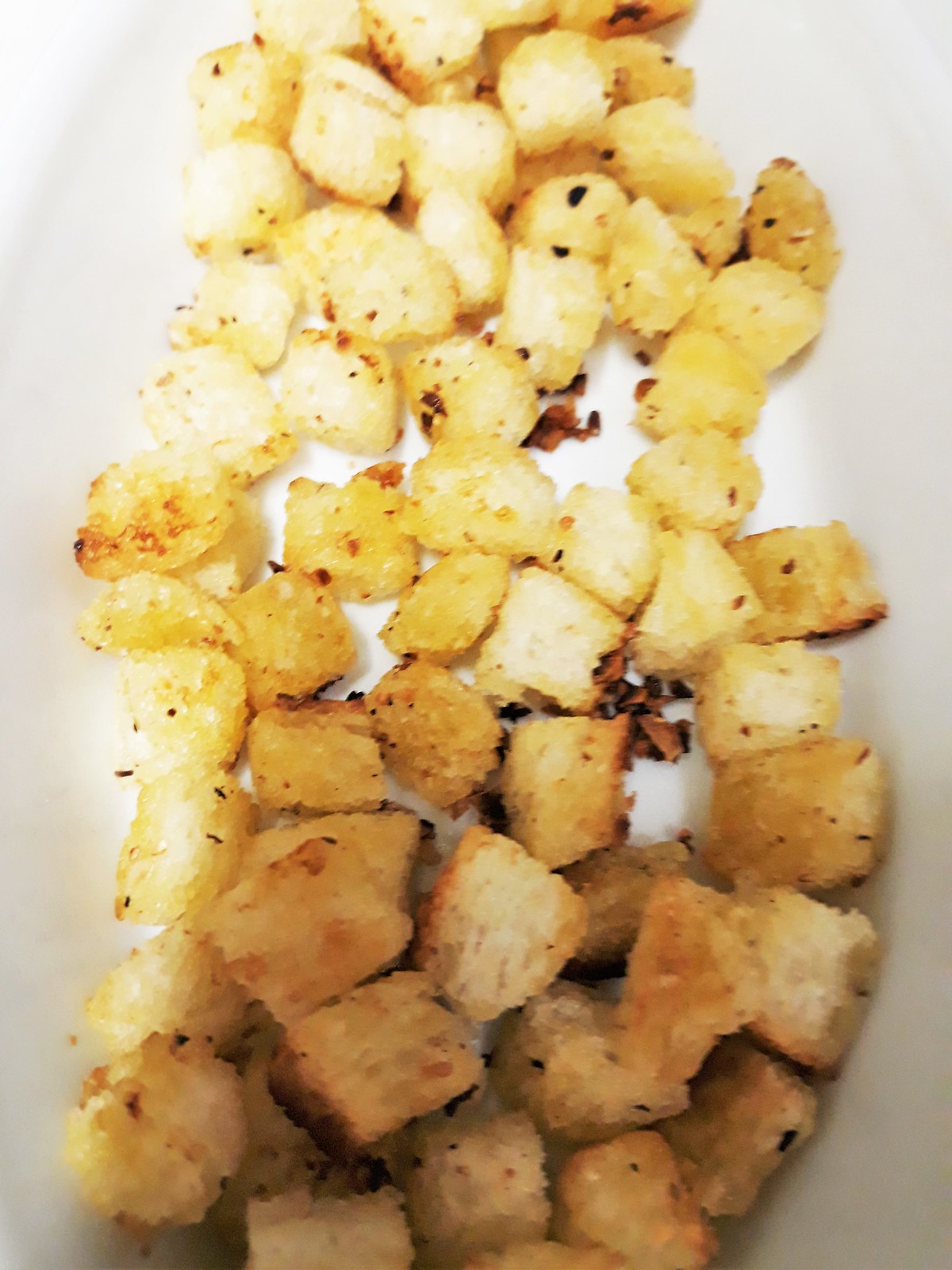This image features a close-up of toasted bread cubes, potentially croutons, captured against a background that transitions from grayish-brown at the bottom to light gray and white at the top. The background subtly suggests the outline of a large white object, possibly a plate or container, enveloping the food. The bread cubes display a variety of tones: towards the upper section, they are lighter yellow with hints of golden brown, likely due to focused lighting. As they progress further down, they become darker and more tan, interspersed with golden brown and some black and brown spots, giving them a toasty appearance. The bread, likely made from white bread, such as French or artisan varieties, shows specks of seasoning throughout, with visible black and brown spots indicating possible spices or sesame seeds, and a trace of red, suggesting a sprinkle of paprika. The scene conveys a mix of textures and flavors, hinting at a seasoned appetizer or salad topping.